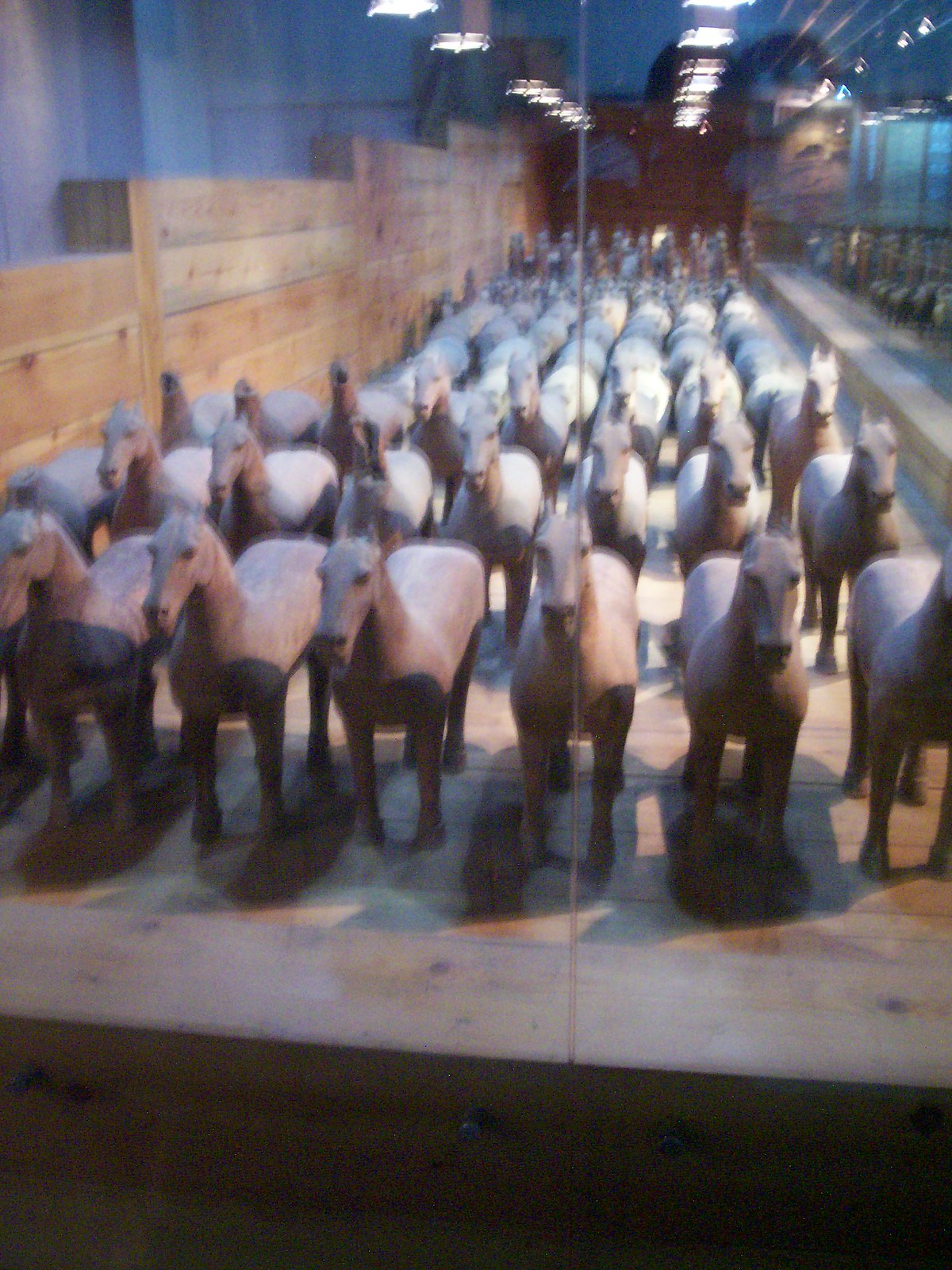The image depicts a blurry, dimly lit scene of numerous horse statues lined up in a display case, viewed through glass. The statues appear to be sculpted and lifelike in scale, possibly made of wood or ceramic, with grayish-brown coloring. Each statue is meticulously arranged in neat rows, stretching out towards the back and left of the image, with some appearing headless. The scene has about eight columns and around 10 to 12 rows of horse statues. Reflective lights from above cast shadows, creating a dark ambiance with a blue tint. The horses stand on a wooden floor, with the backdrop featuring a wood-paneled wall that transitions into blue at the upper section, suggesting a factory-like setting for crafting these life-sized figures. The overall photo is low in contrast and vibrancy, enhancing the mysterious and somber tone of the display.